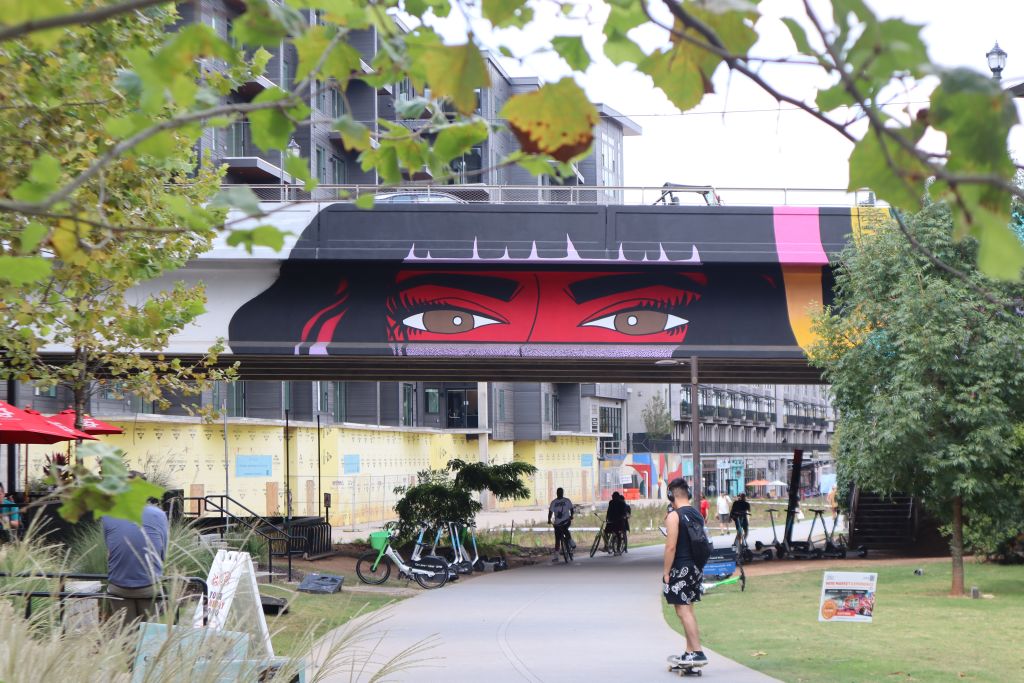The image depicts a vibrant urban park beneath a bridge adorned with striking graffiti art, showcasing the brown eyes, black hair, and red face of a cartoonish woman. The park features a curving pathway lined with green grass and shaded by large trees, with branches and leaves visible at the top of the image. A teenager wearing black shorts, a tank top, a backpack, and headphones rides a skateboard along the path. To the right of him stands a sign on the grass, its details unclear. In the background, several boys ride bicycles toward the viewer, and a row of rentable scooters lines the side. On the left, a man in a blue shirt and green pants sits on a black railing near a set of stairs, possibly leading to an outdoor restaurant with red umbrellas. Beyond the bridge, there are apartment buildings with balconies, adding to the urban landscape. This lively scene is bathed in bright, overcast light, highlighting the interaction between city life and natural elements.